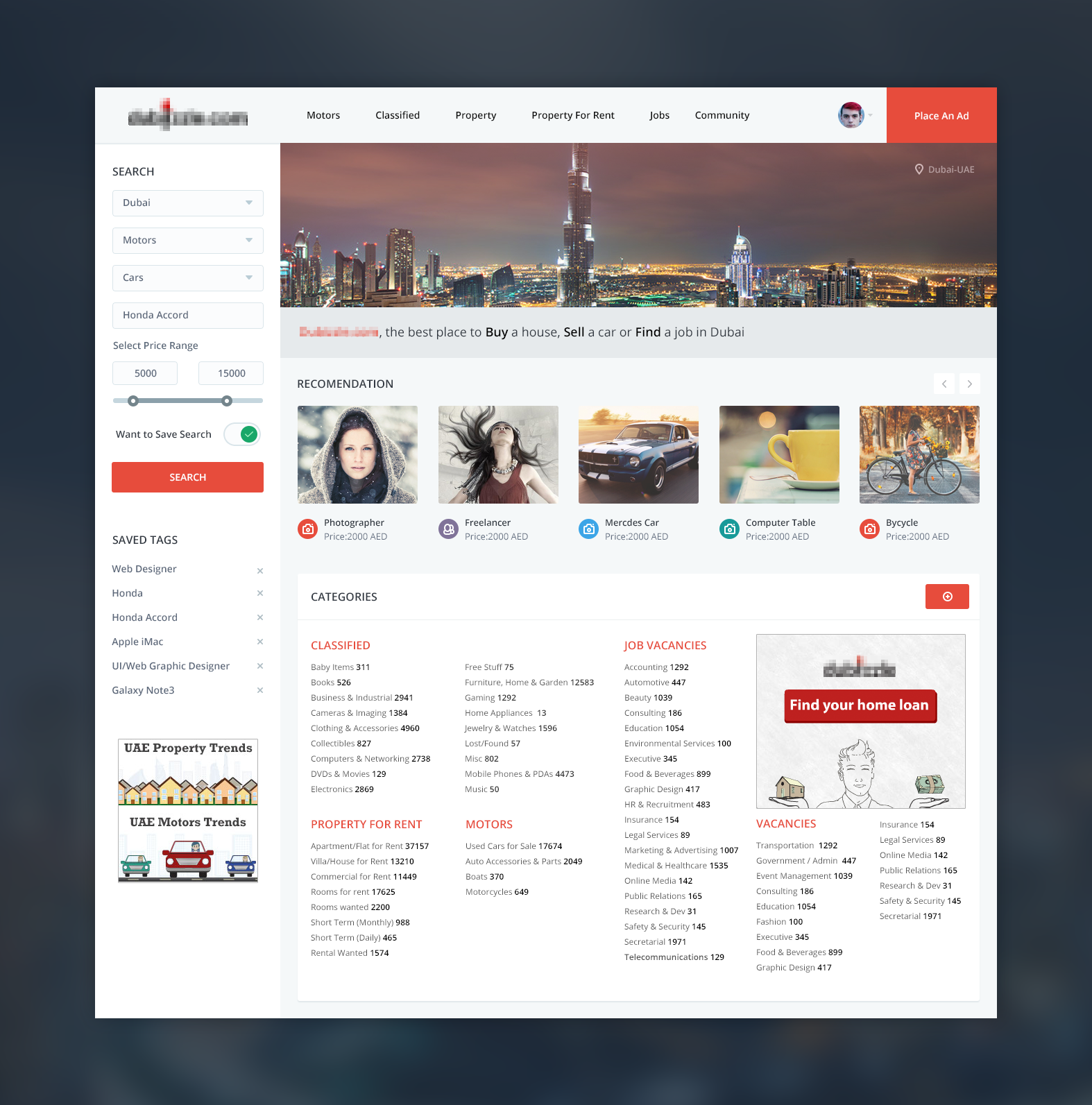The image depicts a classified advertisement website interface specifically tailored for Dubai. At the top of the page, several categories are listed: "Motors," "Classified," "Property," "Property for Rent," "Jobs," and "Community." A prominent red button on the right side invites users to "Place an Ad."

On the left-hand side, a search bar allows users to filter listings. It includes pre-filled fields such as "Dubai," "Motor," "Cars," "Honda," and "Accord." Users can also set a price range from $0 to $5,000 and have an option to save their search. The "Search" button is located just below these options.

The top section of the page is labeled "Recommendations" and features several images and listings. The first recommendation showcases a lady in a sweater with her head covered. The second listing is a freelance service priced at 2,000 AED, accompanied by an image of a woman with dark hair in a red dress, her head tilted back. 

Next is an image of a "Mercedes Car," also priced at 2,000 AED. Following this, a "Computer Table" listing includes a picture of a coffee cup and is priced similarly at 2,000 AED. Lastly, there is a listing for a "Bicycle" with the same price.

Finally, the image reiterates the various main categories, including "Classified," "Properties for Rent," and "Motors," ensuring users can easily navigate through different sections of the site.